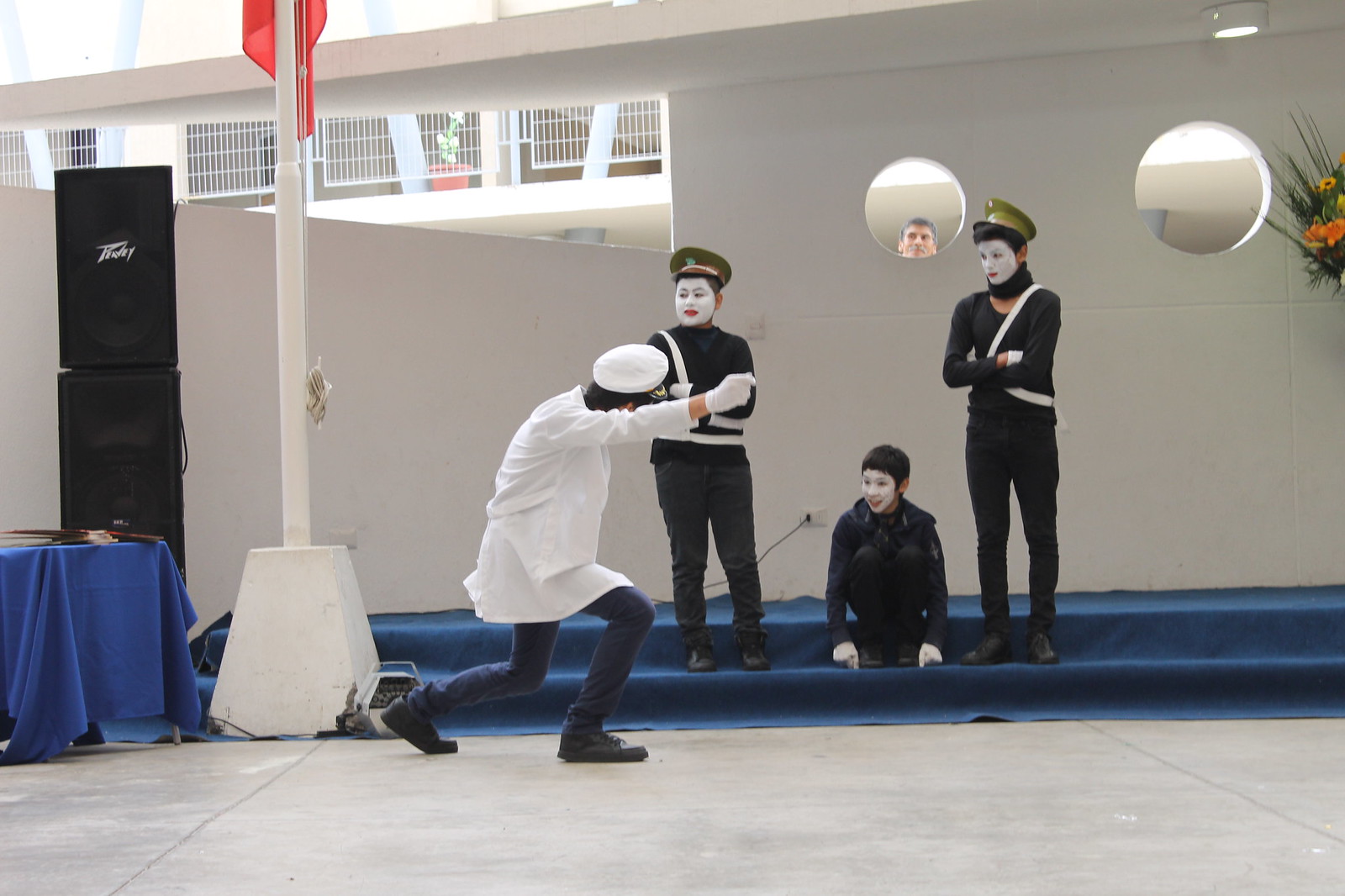In this detailed photograph, a captivating scene of four mimes is captured against a stark white wall featuring two circular windows. Through one of these windows, an observer watches the mimes, adding an intriguing element to the composition. Three of the mimes, with their faces painted white and clad in black outfits trimmed with white, stand on blue stairs, all donning white gloves. The two standing mimes also wear black hats, while the third mime kneels between them. Facing this trio is the fourth mime, distinctively dressed in a white coat, white hat, black pants, and white gloves, who adopts an engaged pose. To the left of the group stands a white flagpole with a partially visible red flag. Adjacent to the flagpole, a table draped in a blue tablecloth supports a tower of black speakers plugged into the wall. The image, meticulously detailed, suggests an indoor performance where the mimes, possibly portraying figures of authority, draw viewers into their enigmatic act.